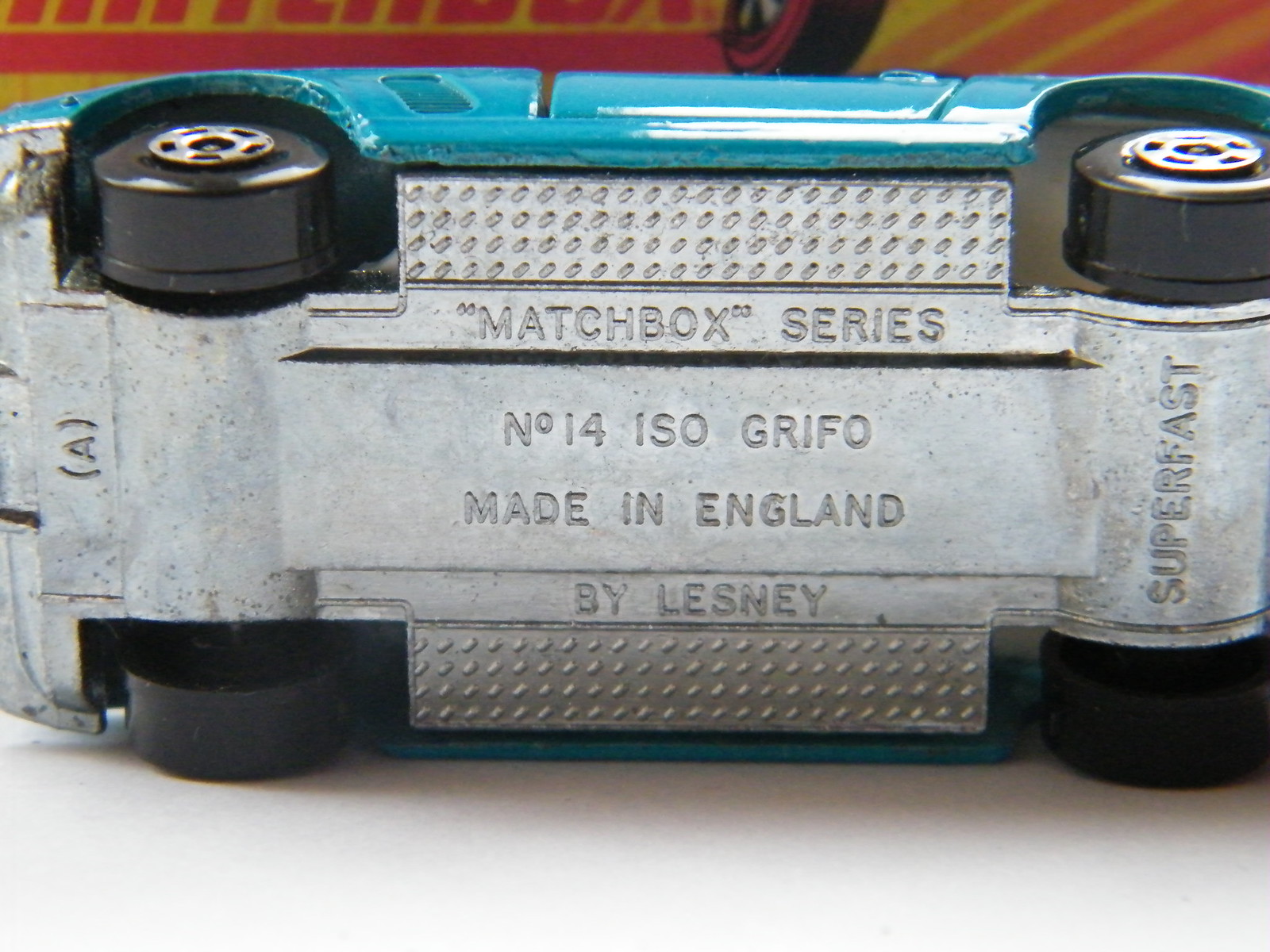The image features a detailed view of a vintage Matchbox toy car, tilted on its side to reveal the underside. The car, likely a turquoise or teal color, shows minimal visible portions of the door and fenders and rests on a stark white tabletop. The bottom, made of a silver-gray metallic material, displays raised text with the following information: "Matchbox Series," "Number 14," "ISO GRIFO," and "Made in England by Lesney." An "A" in parentheses is located by the back axle, and "Superfast" is mentioned near the front wheels. The four black wheels are visible, including two hubcaps. The background partially shows a poster, predominantly in orange and yellow or possibly red, depicting a cut-off wheel design, suggesting an older image of a Matchbox-related advertisement.